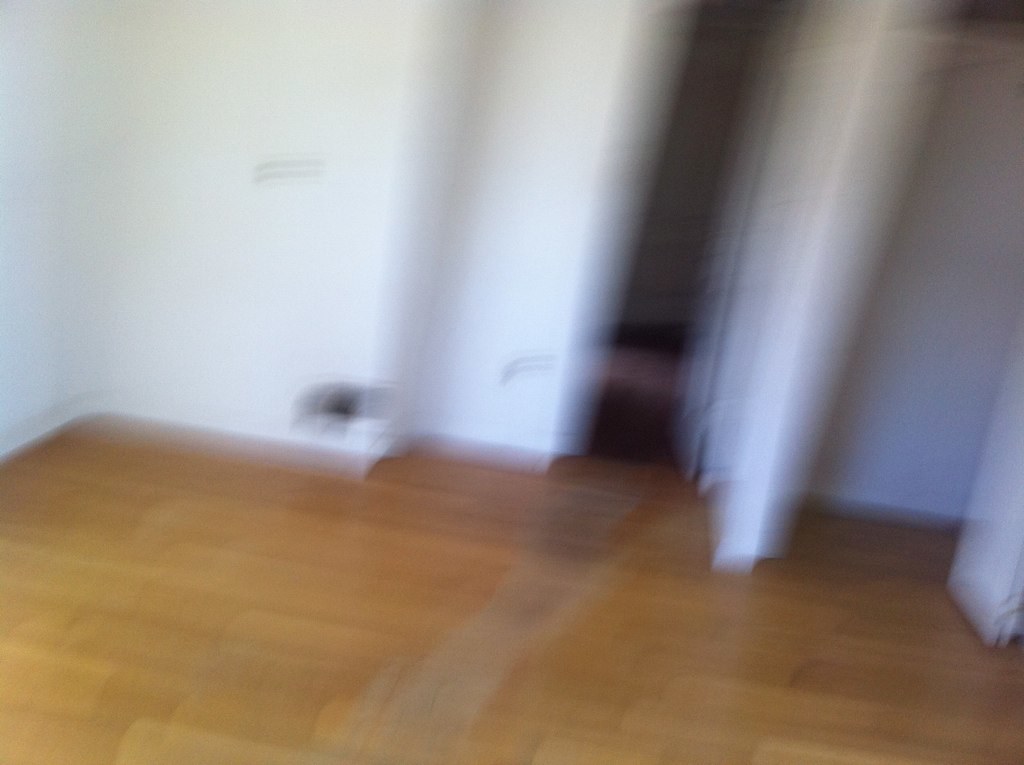The image is a highly blurred photograph of a brightly lit, empty room with light brown, shiny wooden floors. The floor has a noticeable worn area in the middle, appearing lighter beige against the oak finish. White baseboards line the walls, which are entirely white and feature some black marks. On the right side, there is a small closet with bifolding doors that are slightly open, revealing a dark interior. To the left of this closet, the wall jags in and out, suggesting it could be an alcove, though the space is ambiguously defined due to the blurriness. Additionally, an open white door, possibly leading to another room or a bathroom, can be seen in the background. The overall space seems to suggest a non-kitchen room, potentially a bedroom.